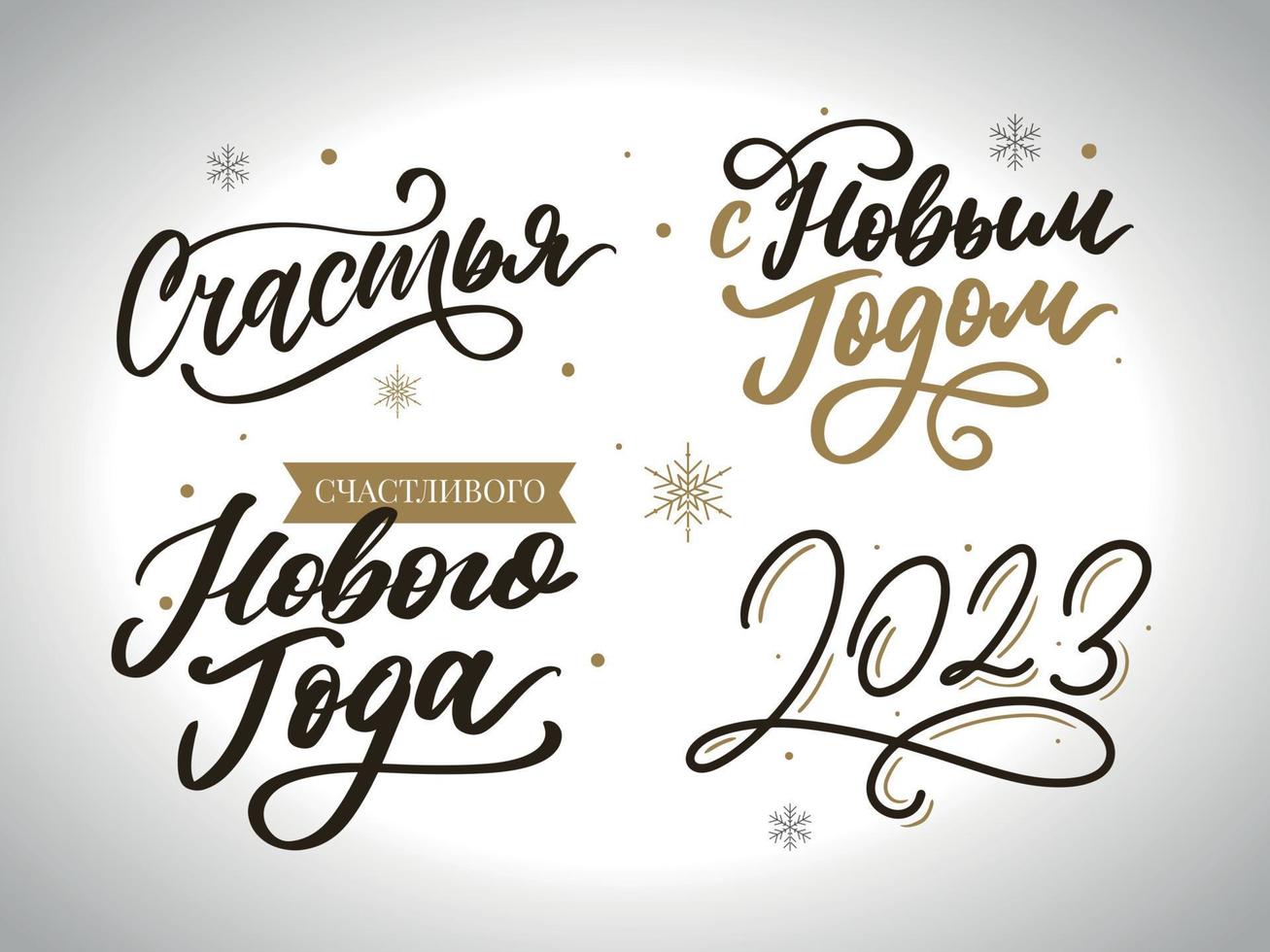The image showcases a festive card, likely for Christmas or New Year. It features a white backdrop with the corners transitioning into a darker gray. Within the background is a brighter white circle. The card is adorned with writing in a curved cursive-like font that does not appear to be in English, possibly in a foreign language or using unrecognizable words. Part of the text in the lower left corner sits beneath a small banner, which has more text and looks like it might contain Russian characters. In the upper right corner, the text is divided into black and gold words. The bottom right highlights the year "2023" in a decorative, curling font. Scattered throughout the design are images of stylized black and gold snowflakes and numerous gold and silver dots, adding a festive touch to the card.